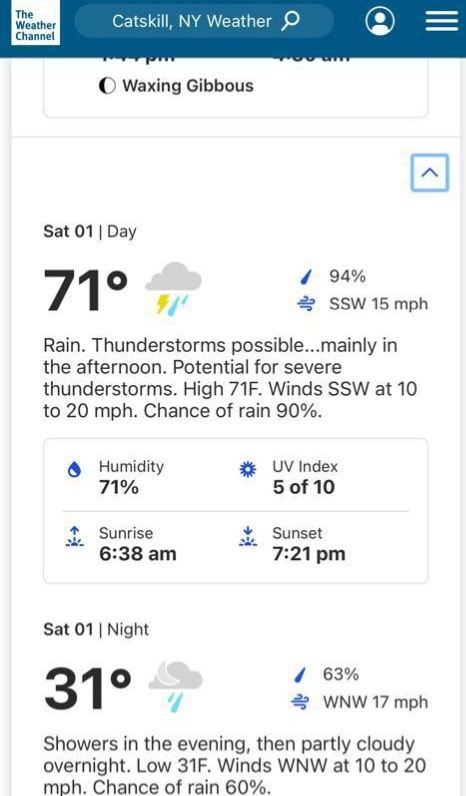This is a detailed screenshot of The Weather Channel's mobile app, captured and cropped. The image showcases the app's interface designed with a dark blue header at the top. On the left side of the header, the Weather Channel logo is prominently displayed. Centrally placed in the header is a search bar containing the text "Catskill New York Weather." To the right of the search bar, there are two icons: a profile icon and a menu icon represented by three horizontal lines.

Just below the header, the app's body transitions to a white background. At the very top of this section, the faint edge of an image depicting a moon phase is visible, indicating the previous day's forecast. Immediately below, it provides details for the forecast on Saturday. The exact month is not specified, but the date is clearly marked as "01."

A large numerical display shows the temperature as 71 degrees in bold black characters. To its right, there is a weather icon depicting a cloud with rain and lightning, symbolizing stormy weather. Farther to the right is a detailed precipitation chance, marked as 94%. A wind icon is present as well, indicating wind conditions from the south-southwest at 15 miles per hour.

Following the icons, the narrative part of the forecast states: "Rain, thunderstorms possible, mainly in the afternoon. Potential for severe thunderstorms. High 71 degrees. Wind south-southwest at 10 to 20 mph. Chance of rain 90%."

Below this detailed forecast, a small box offers additional weather information, including humidity levels, UV index, times for sunrise and sunset.